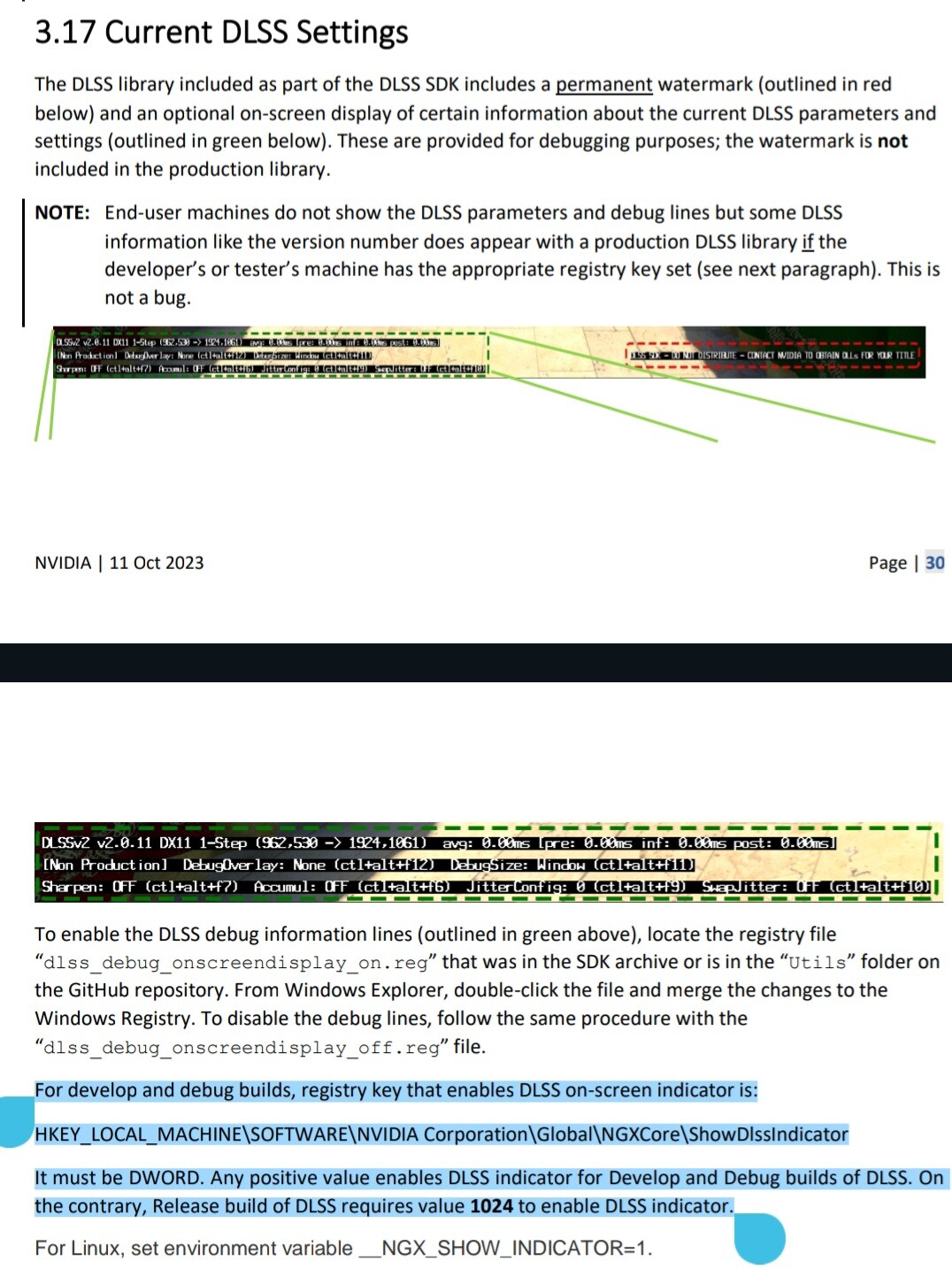This image displays current DLSS settings, prominently featured in the upper left corner with the label "3.17 Current DLSS Settings". Below this title, there is a paragraph explaining that the DLSS library, part of the DLSS SDK, includes a permanent watermark (outlined in red) underneath an optional on-screen display for certain information regarding the current DLSS parameters and settings (outlined in green). The image appears to contain two stacked paragraph sections. The bottom section includes a highlighted blue portion indicating "DLSS Off" with a registry key for development and debug builds. The specific Windows registry address is provided, noting that it must be a DWORD value, with any positive value enabling the DLSS indicator for these builds.